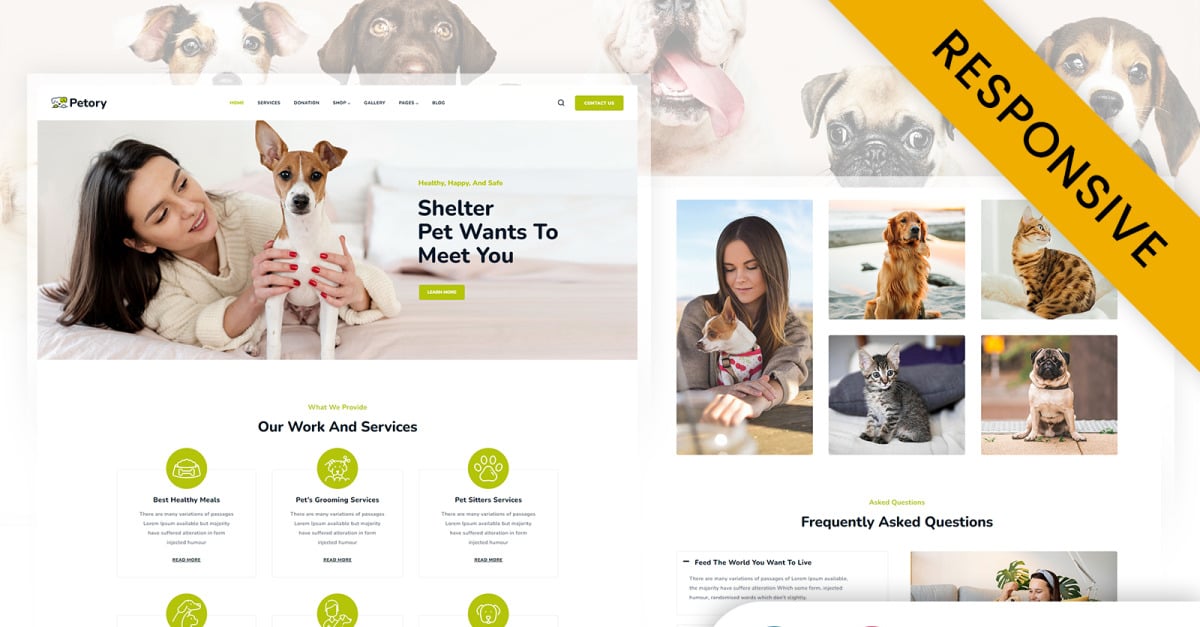The website interface features a prominent navigation bar across the top, displaying five different dogs in various poses. The central image is a close-up shot of a dog's mouth with its tongue playfully hanging out. To the right, the website’s name "Pettery" is boldly displayed. Below the navigation bar are six clickable options alongside a search icon represented by a magnifying glass.

An attention-grabbing image to the left depicts a woman lounging on a bed, cradling a cute dog with one ear up and one ear down. She gazes affectionately at the dog, which is held gently with her hands around its chest. The image is overlaid with the text "Shelter pet wants to meet you," inviting users to learn more about adoption opportunities.

The section titled "Our Work and Services" showcases six offerings: best healthy meals, pet grooming services, and pet sitting services. Each service is represented by a distinct green icon; however, the icons for the bottom three services are partially obscured and not fully visible.

To the right, images of cats, dogs, and a woman working at her computer with her dog in her lap create a warm and engaging atmosphere. This section includes a Frequently Asked Questions (FAQ) section, addressing common user inquiries.

A gold diagonal banner stretches from the top-left to the bottom-right of the screen, adorned with black lettering that reads "Responsive," emphasizing the website's adaptability and user-friendly design.